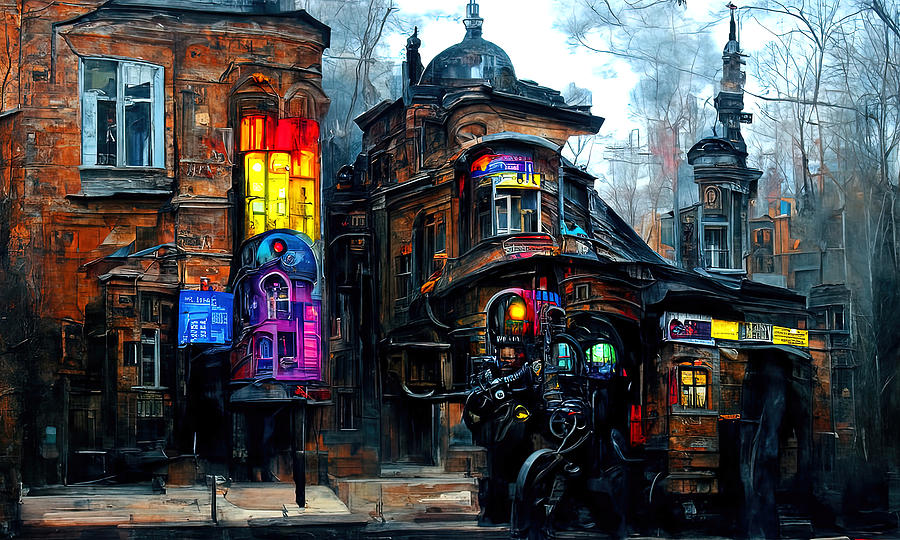This artwork depicts a richly detailed artist's vision of a Victorian steampunk city, blending futuristic and retro elements with precision. The image showcases multiple brick and vividly colored buildings, most notably, a prominent two-story structure on the left with a curved corner resembling a turret, adorned with stained glass windows and exposed piping. A central brown building, reminiscent of a log cabin with green and black windows, contrasts against the urban scenery. The sidewalk below shows signs of wear, featuring brick sections that appear eroded. In the scene, a machine akin to a double-decker bus, complete with spindles, gears, and pipes, adds to the intricate Victorian steampunk aesthetic. The sky overhead is a muted gray with dark clouds, enhancing the dark tones of the picture while bright hues offer a striking contrast. Bare trees stretch upwards, and distant structures with large, rounded roofs and cathedral-like steeples add depth. Scattered around are ambiguous figures that might be droids, adding to the city's bustling yet mysterious atmosphere.